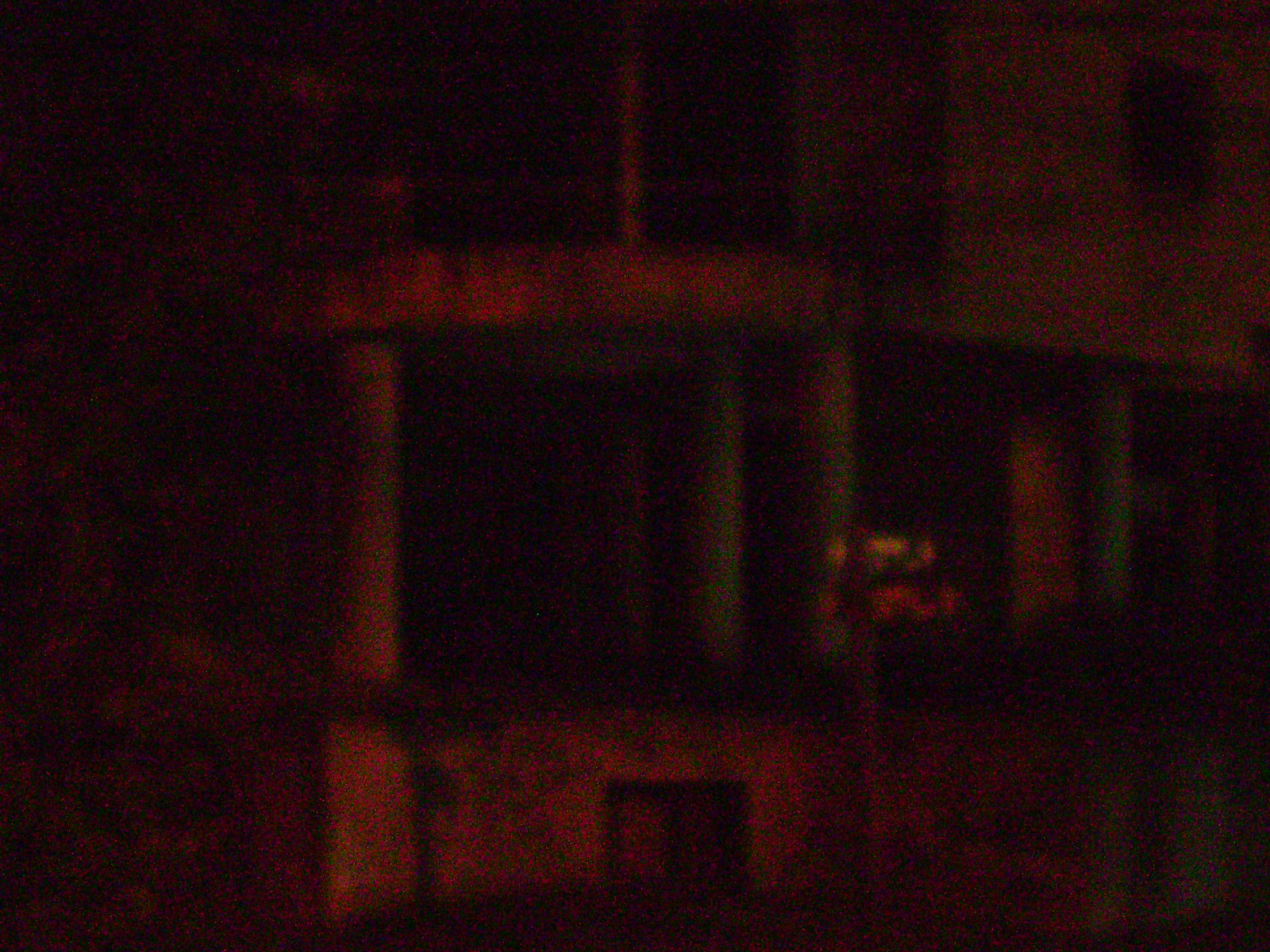A dimly lit image reveals the vague outline of a mysterious structure. The scene is shrouded in darkness, save for sparse red lighting that highlights various objects scattered in the foreground. These objects mostly consist of cubic forms, suggesting a constructed environment. Positioned near the center are tube-shaped columns, their cylindrical forms subtly illuminated by the ambient light. Intriguingly, red and yellow lines trace across the image, possibly indicating lens flare or other reflective surfaces. Towards the bottom of the frame, a doorway becomes visible, marking an entry point into the large, blocky edifice. Above this threshold, the silhouette of an upper floor with possible openings hints at further architectural features. Despite the obscurity, the image evokes a sense of depth and complexity, leaving the true nature of the structure open to interpretation.